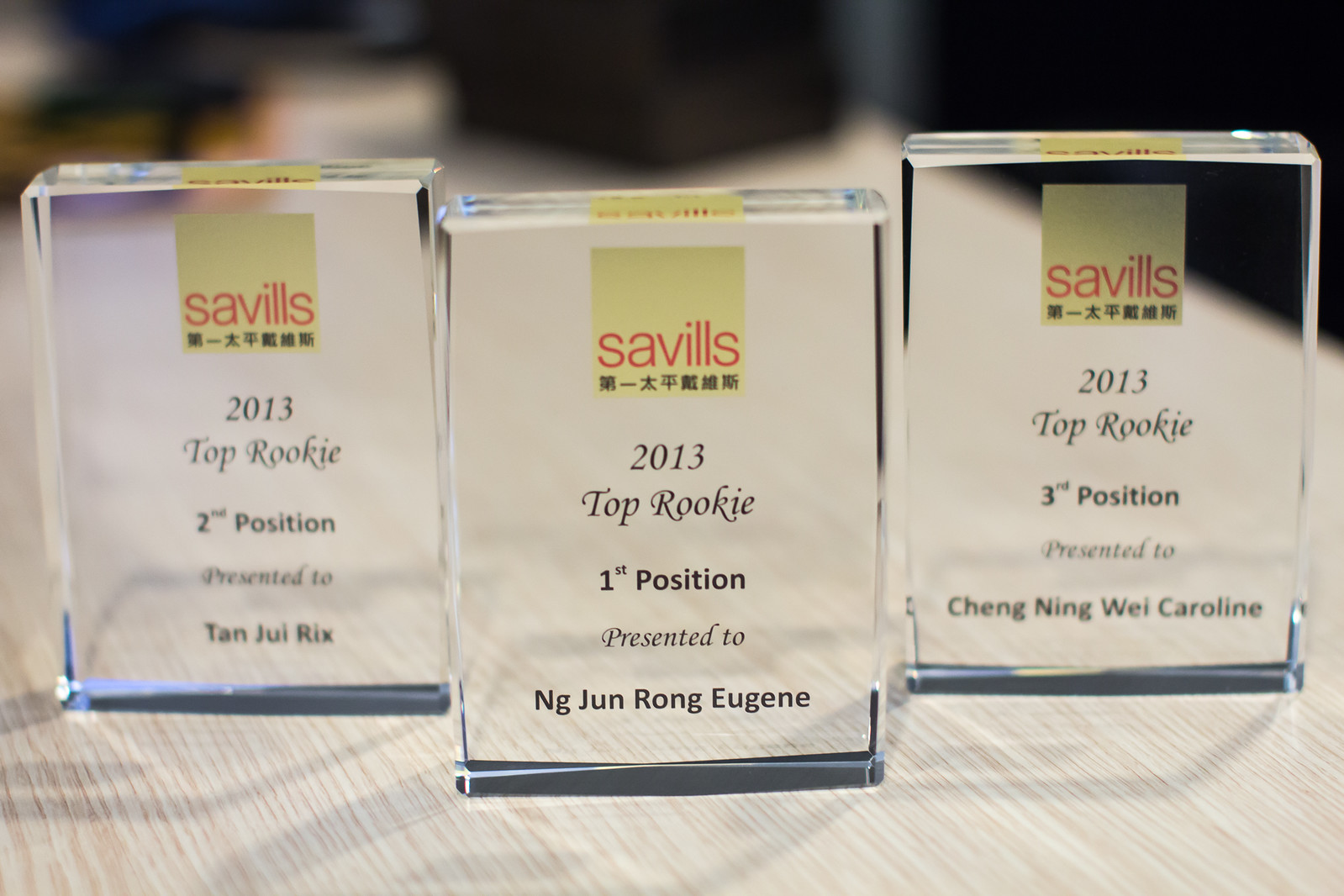This color photograph, taken in landscape orientation, captures three clear glass award plaques neatly arranged side by side on a pale brown, wooden-grained table. These plaques are vertically oriented rectangles and each features a logo at the top in red type on a yellow background that spells out "SAVILLS." Beneath the logo, there is a line of text in black Chinese characters. Below these characters, each plaque displays the year "2013" followed by the title "Top Rookie," and the respective positions. The center plaque, slightly in front of the others, reads "1st Position" and is presented to NG Jun Rong Eugene. The plaque on the left, slightly behind, reads "2nd Position" and is presented to Tan Ju Ri. The plaque on the right, also slightly behind, reads "3rd Position" and is presented to Chang Ning Hui Caroline. Each name is prominently displayed in black print on the clear glass surface.